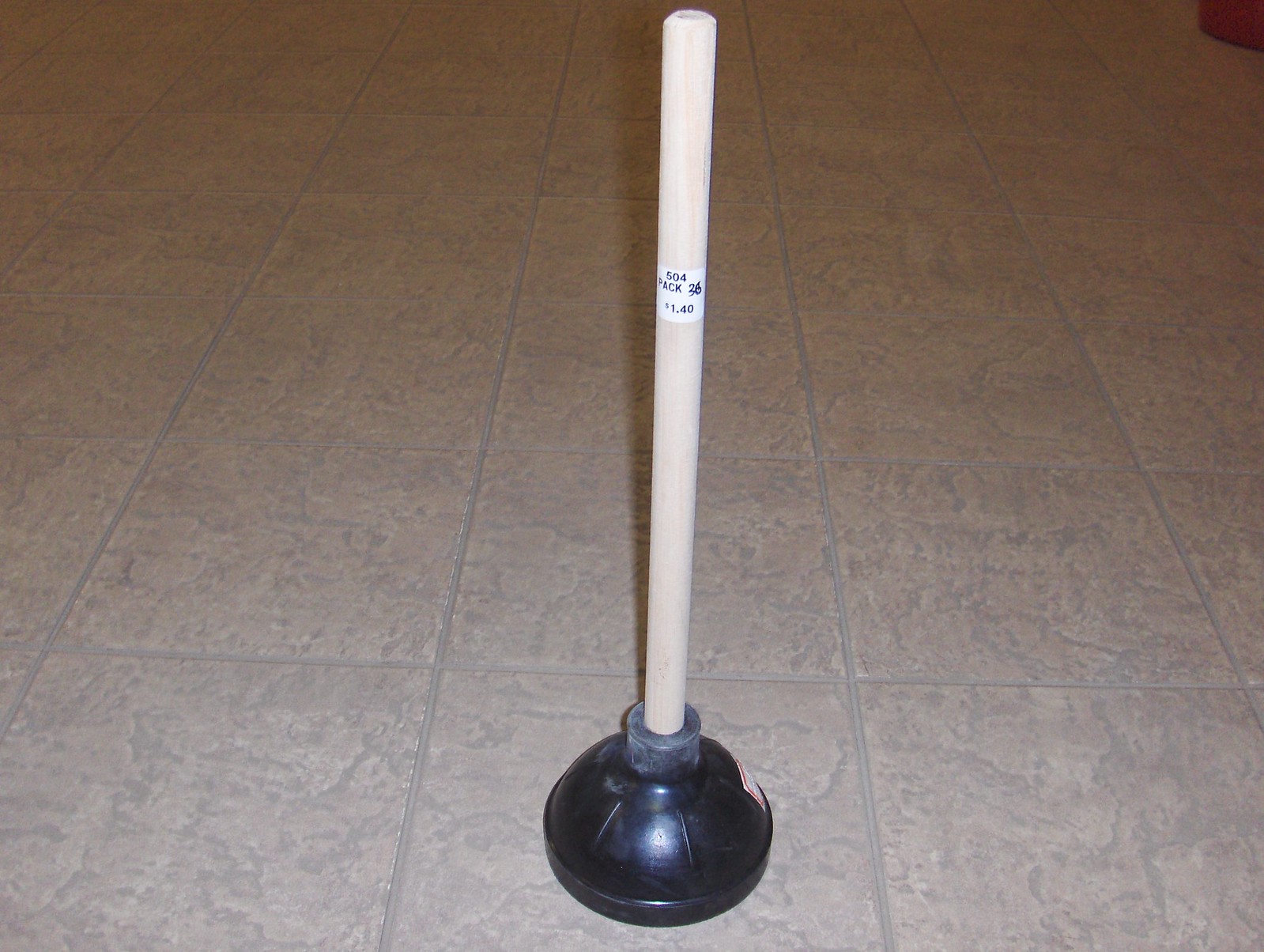This detailed image depicts a typical toilet plunger prominently positioned on a tiled floor. The floor tiles are square, exhibiting a light tan or brown color with a slightly textured, aged appearance and possibly a tan or gray grout. The plunger, which features a wooden handle and a black rubber or plastic base, stands upright in the middle of one of the tiles. A small white price tag with black text can be seen near the top of the handle, indicating "504 Pack" and a price of "$1.40". Additionally, there is a noticeable white and red warning label on the right side of the plunger. Despite the worn look of the tiles, the plunger itself appears quite shiny, suggesting it may be recently cleaned, although some dust is visible on the top of the handle.